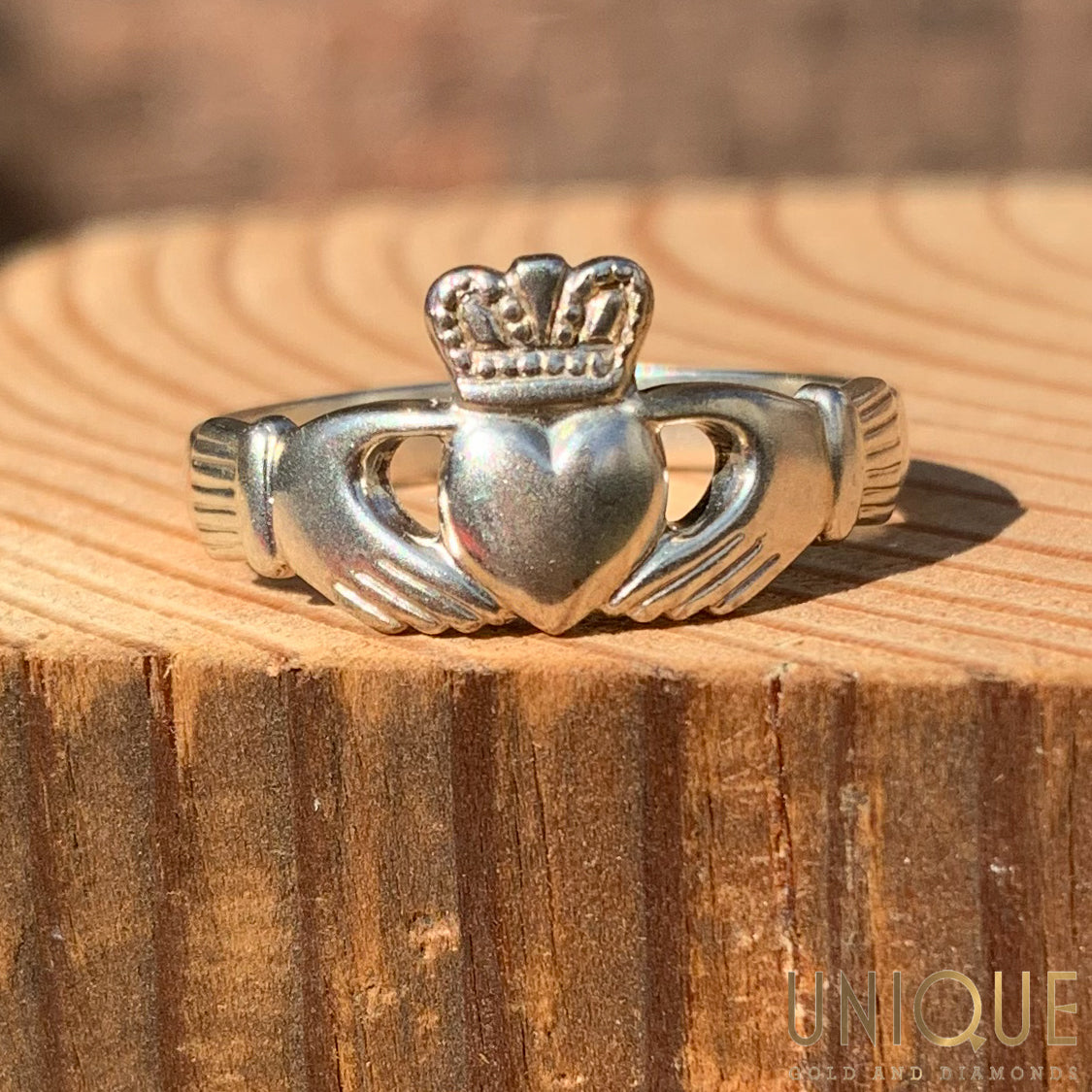This image, taken outdoors, showcases a silver ring displayed on a carved tree stump with distinct grooves. The stump features a mix of darker and lighter browns, with a flat, grooved surface on top. In the bottom right corner, the text "Unique Golden Diamonds" is elegantly inscribed in gold. The centerpiece of the image is the silver ring, meticulously designed with two hands caressing a heart topped with a crown. The textured cuffs of the hands suggest they are adorned with sweater-like details. The ring, possibly slightly tarnished, glistens slightly, highlighting its intricate design and potential sentimental value, likely intended for a loved one.